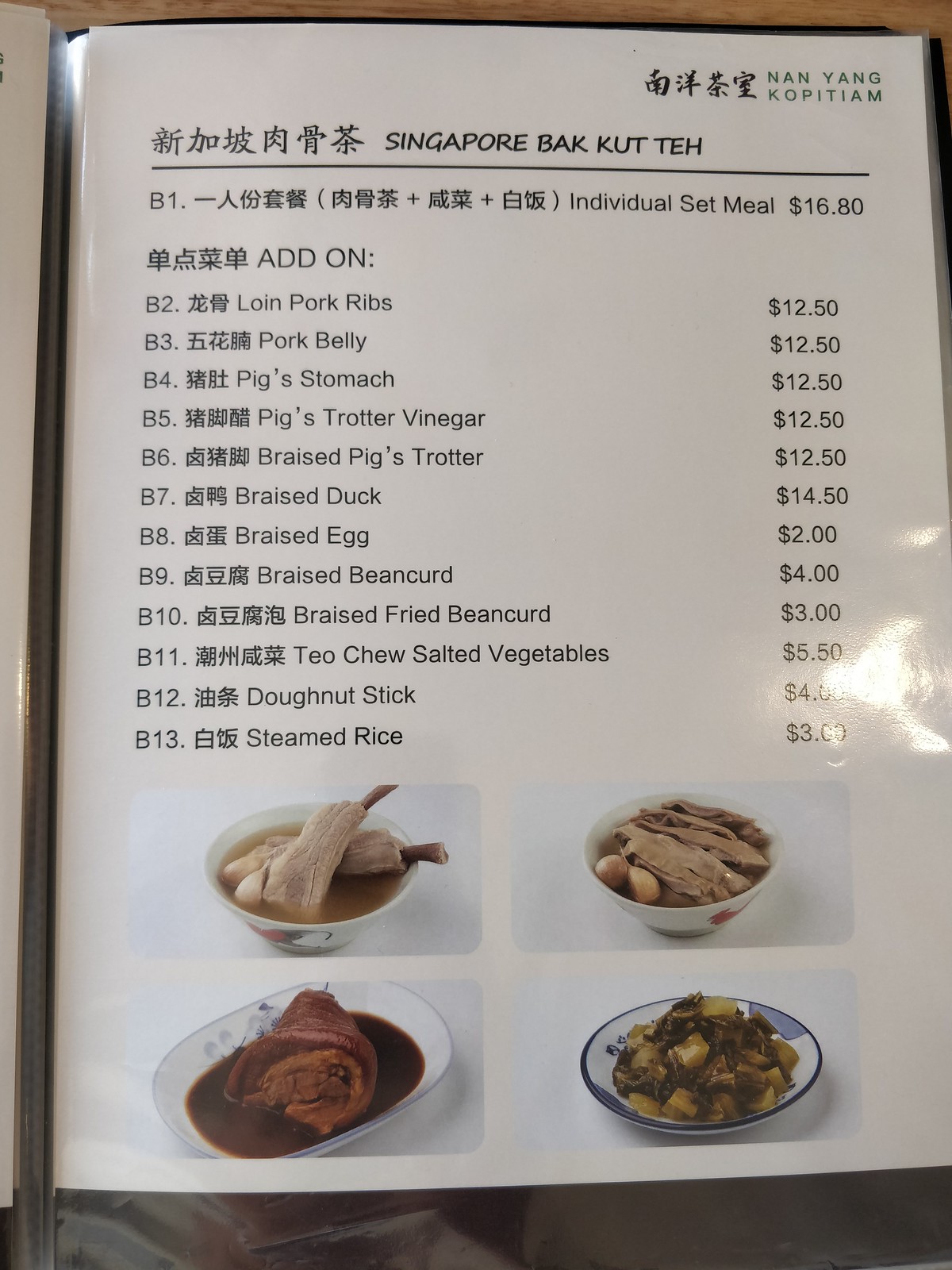This image is a high-resolution photograph of a restaurant menu taken in portrait mode, making the image taller than it is wide. The background subtly features part of the table, providing context to the dining setting. The menu prominently displays various Asian characters, indicative of the regional cuisine. At the top of the menu, "Singapore Bak Kut Teh" is written, suggesting that the restaurant specializes in this traditional Singaporean dish.

The menu is organized with different sections detailing set meals and add-ons. The "Individual Set Meal" is priced at $16.80, with a description in both English and an Asian language. An array of add-ons is listed below this, each accompanied by its name in English, a corresponding Asian character, and its price. These add-ons range from options like "Loin Pork Ribs," "Pork Belly," and "Pig's Trotter Vinegar" to "Braised Duck," "Braised Egg," "Braised Bean Curd," and more. The prices for these items vary, spanning from $2.00 to $14.50.

At the top right corner of the menu, the restaurant's name, "Nanyang Kopitiam," is displayed, suggesting a connection to traditional Singaporean coffee shops. The very bottom of the menu showcases images of four different bowls, each filled with various dishes offered by the restaurant, providing a visual preview of the cuisine.